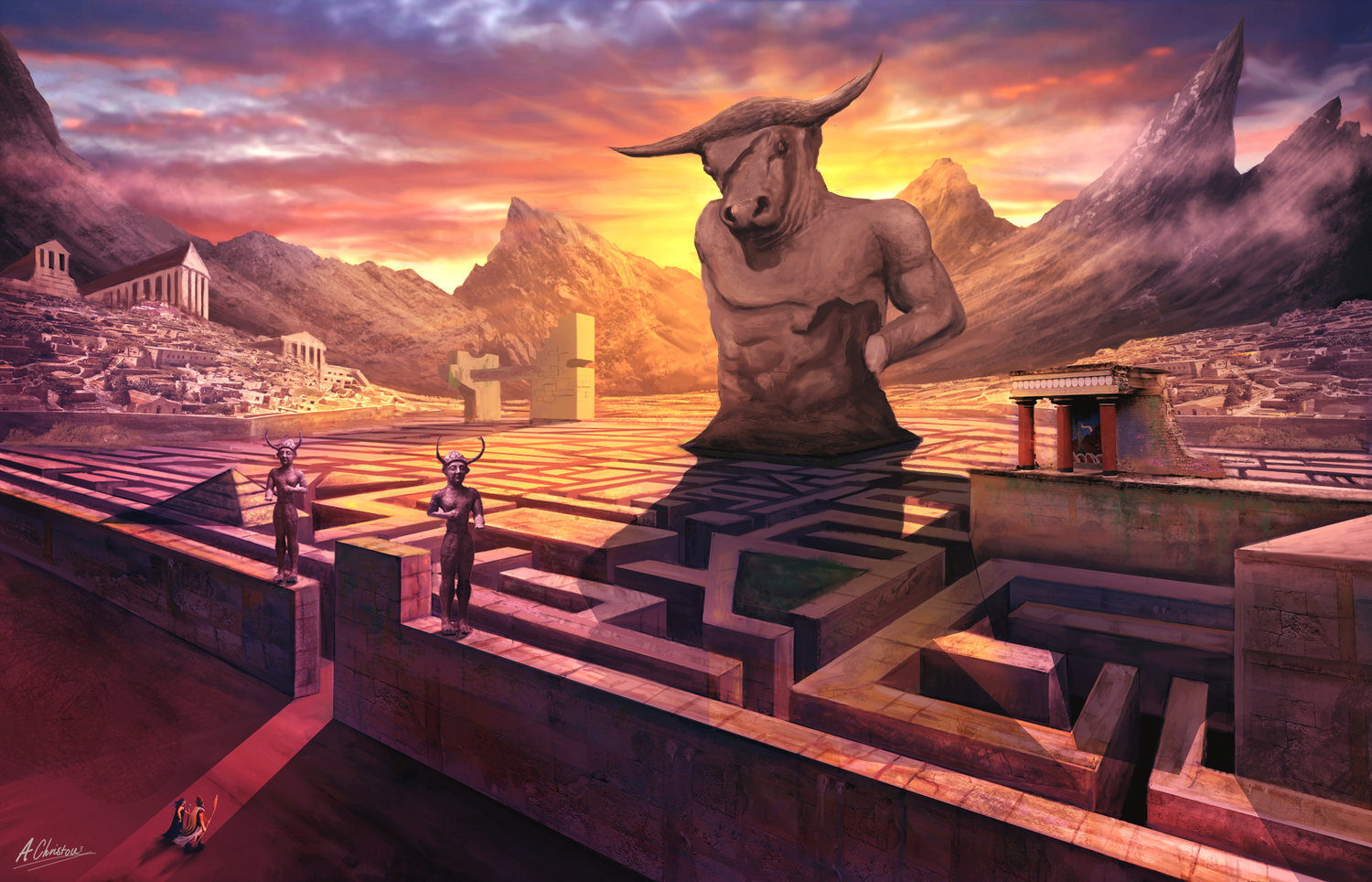This piece of artwork, possibly a digital illustration or painting, depicts a vivid fantasy scene inspired by the ancient Greek myth of the Minotaur. Dominating the center of the image is a colossal stone Minotaur statue, notably missing its right hand, with the left arm visible up to the forearm, but also missing the hand. The statue stands towering, seemingly around 50 feet high, making the tiny human figures at the base appear insignificant against its grandeur. These figures are seen entering a labyrinth comprised of imposing stone walls, intricately woven beneath the statue.

The artwork is signed in white at the bottom left corner with a signature that includes "A" followed by a capital "C" and underlined twice. The labyrinth is bathed in light that illuminates the small figures as they navigate its depths. Flanking the entrance are additional Minotaur statues, adding to the scene’s mythical ambiance.

In the background, a series of jagged mountains rise sharply, framing the skyline that transitions through vibrant hues of yellows and oranges, suggesting either a sunrise or sunset. To the left, nestled on a hillside, are ancient structures reminiscent of Greek ruins, enhancing the classical atmosphere of the image. The scene combines elements of both fantasy and ancient history, brought to life with rich, atmospheric detail.